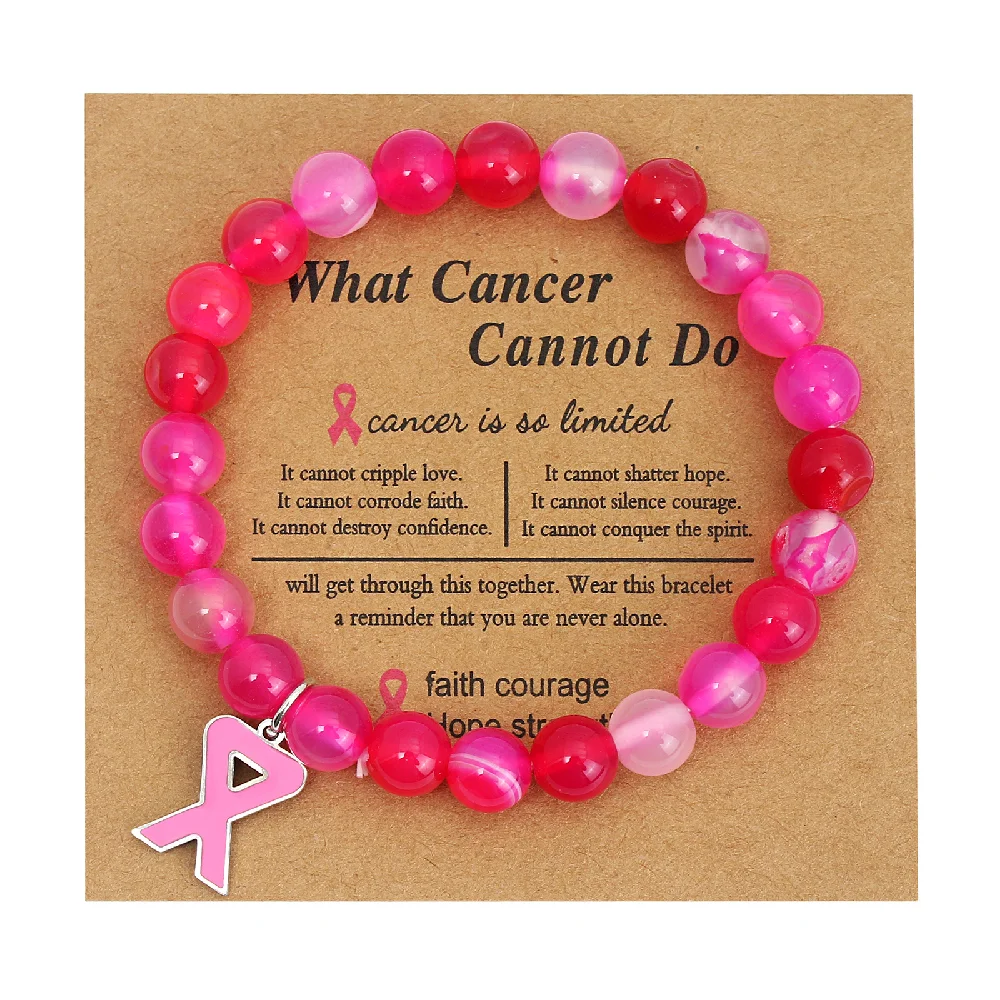The product photograph showcases a delicate beaded bracelet on a square-shaped recycled brown cardboard card. The bracelet forms a perfect circle around the card's black text, which reads: "What Cancer Cannot Do. Cancer is so limited. It cannot cripple love. It cannot corrode faith. It cannot destroy confidence. It cannot shatter hope. It cannot silence courage. It cannot conquer the spirit. We'll get through this together. Wear this bracelet, a reminder that you are never alone." 

The bracelet features beads in varying shades of pink, red, and frosty white, resembling pink and white marbles. A notable charm in the shape of a pink ribbon, symbolizing breast cancer awareness, adorns the bottom left side of the bracelet. The charm has a circle at the top with the ribbon tails extending below. The elegant and thoughtful design of both the bracelet and the card aims to convey hope, strength, and solidarity.